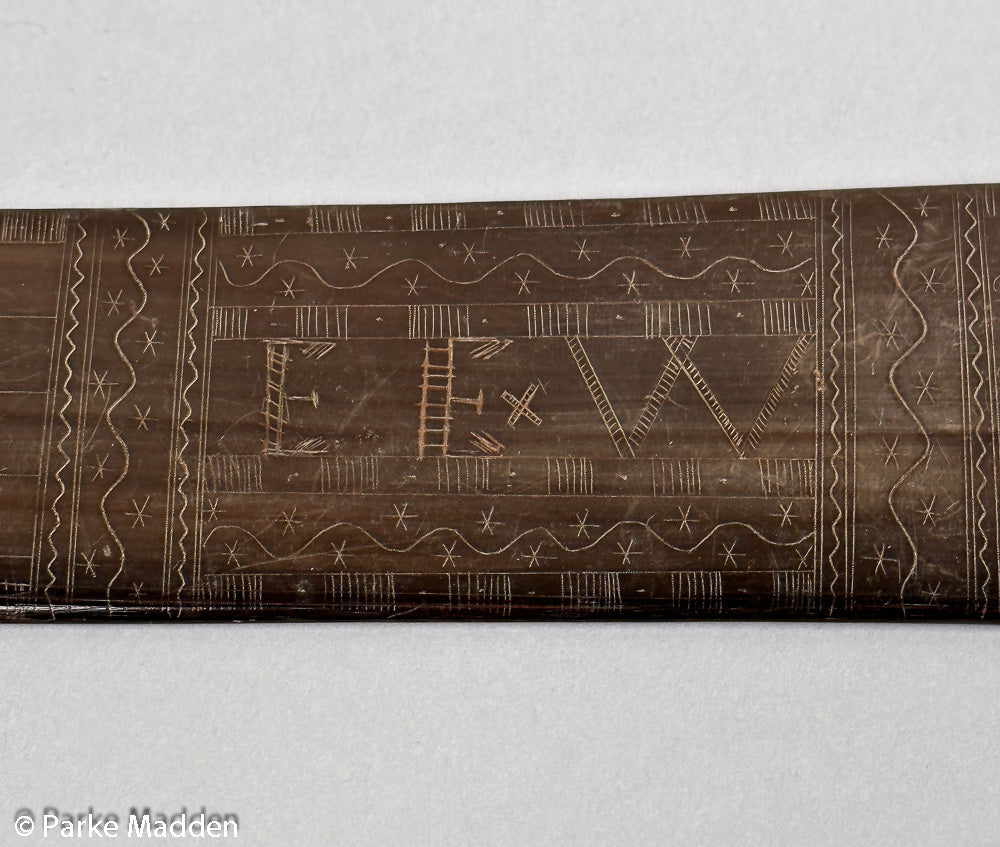The image showcases a detailed etching on a piece of dark-stained wood, possibly teak, with a white background that emphasizes the artwork. The focal point is the intricate carvings on the wood, which highlight a mix of abstract elements. Surrounding the border are wavy lines and crude star shapes, creating a frame-like pattern at the top, bottom, and both sides. Inside this border, rows of vertical lines separated by dots guide the eye toward the center, where a series of ladder-like structures are prominently featured—two upright and four slanted. Centrally etched are the initials "EXW," flanked by the vertical and horizontal lines. The piece is dense with hash marks, squiggly lines, stars, and possibly Xs, woven into a cohesive design that hints at abstract symbolism. At the bottom left corner, the artwork is copyrighted to Park Madden.